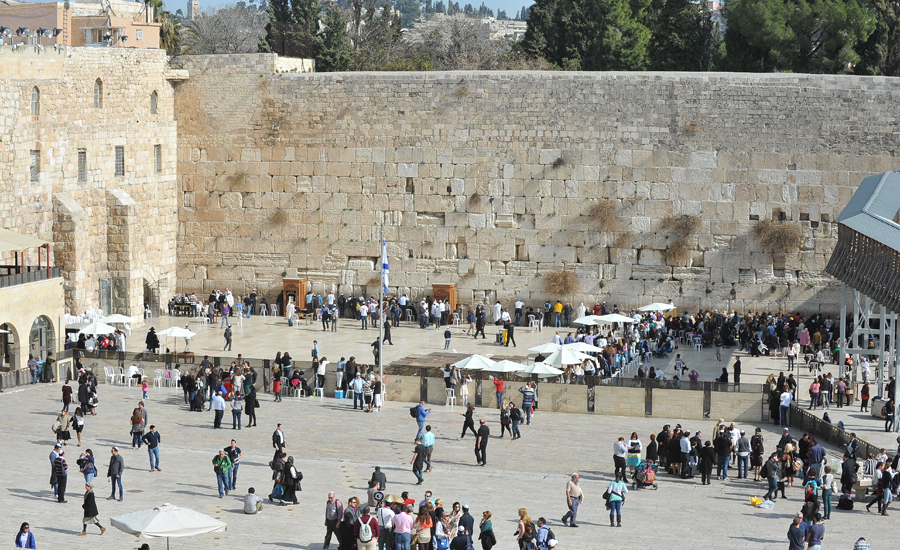This photo captures an ancient, historical site in Israel, featuring the iconic Jewish praying walls, known as the Western Wall, forming the back boundary of a large, entirely concreted courtyard. The image, seemingly taken from an elevated perspective—perhaps a second or third floor—presents thousands of visitors and pilgrims. At the forefront, individuals are seen praying against the massive, towering stone wall, while groups of tourists meander around the expansive square. Scattered tables with umbrellas are visible, possibly for visitors to gather or purchase items. Additional structures and buildings, including ancient stone constructions that might date back to historical times, flank the courtyard. People in the scene appear small due to the photo's vantage point, accentuating the monumental scale of the setting. In the upper background, the skyline reveals more buildings and some sparse greenery, juxtaposing the ancient stone with the modern cityscape. The lack of signage emphasizes the site's raw, historic ambiance, with visitors standing on buckets and chairs peering over gates and fences that segment the space.